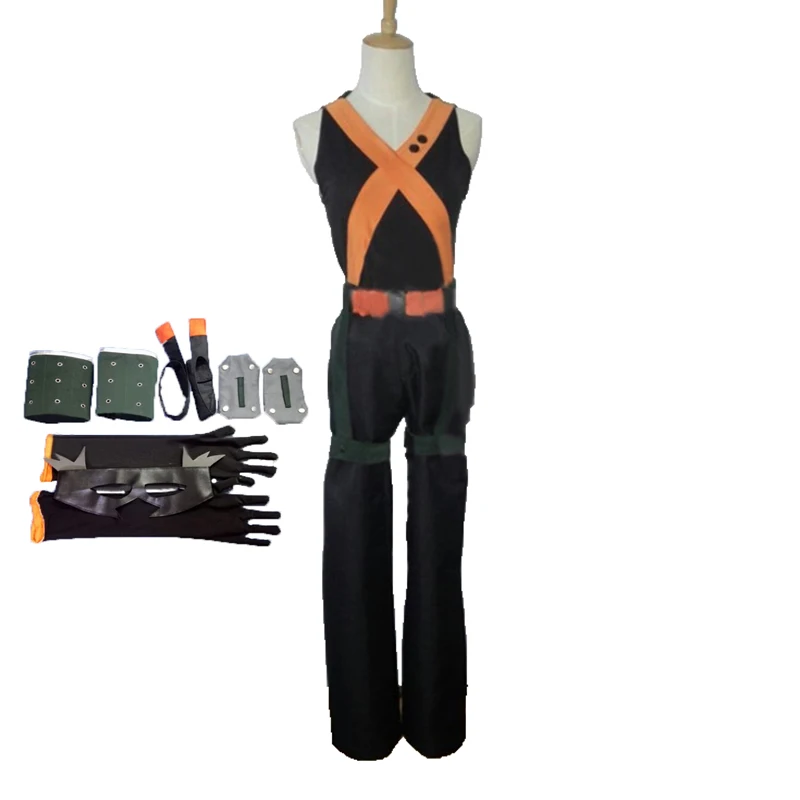The image features a headless and armless mannequin positioned against a plain white background. The mannequin, which is a subtle off-white color, is dressed in a complex cosplay outfit. The sleeveless top is black and forms an orange X across the chest, made by two diagonal orange ribbons that intersect, complete with two small black buttons where the ribbons meet on the upper right side. The pants are dark gray and are secured by a distinctive red belt with a dark gray, square buckle. Dark green bands encircle the thighs, adding to the detailed design of the costume.

Alongside the mannequin, to the left, lies an array of accessories that complement the outfit. There are two rows of items: the top row features green wristbands adorned with silver punch holes and what appears to be a dark gray headband with orange tips. Below, there are two long black gloves with orange ends, presumably where the elbows would be, and a black eye mask that has openings for the eyes and nose.

This digital image appears to represent a meticulously crafted cosplay costume, reminiscent of attire from the anime "My Hero Academia," though there is no textual confirmation of this within the image. The overall color palette of the costume and accessories prominently features black, orange, dark gray, and dark green hues.